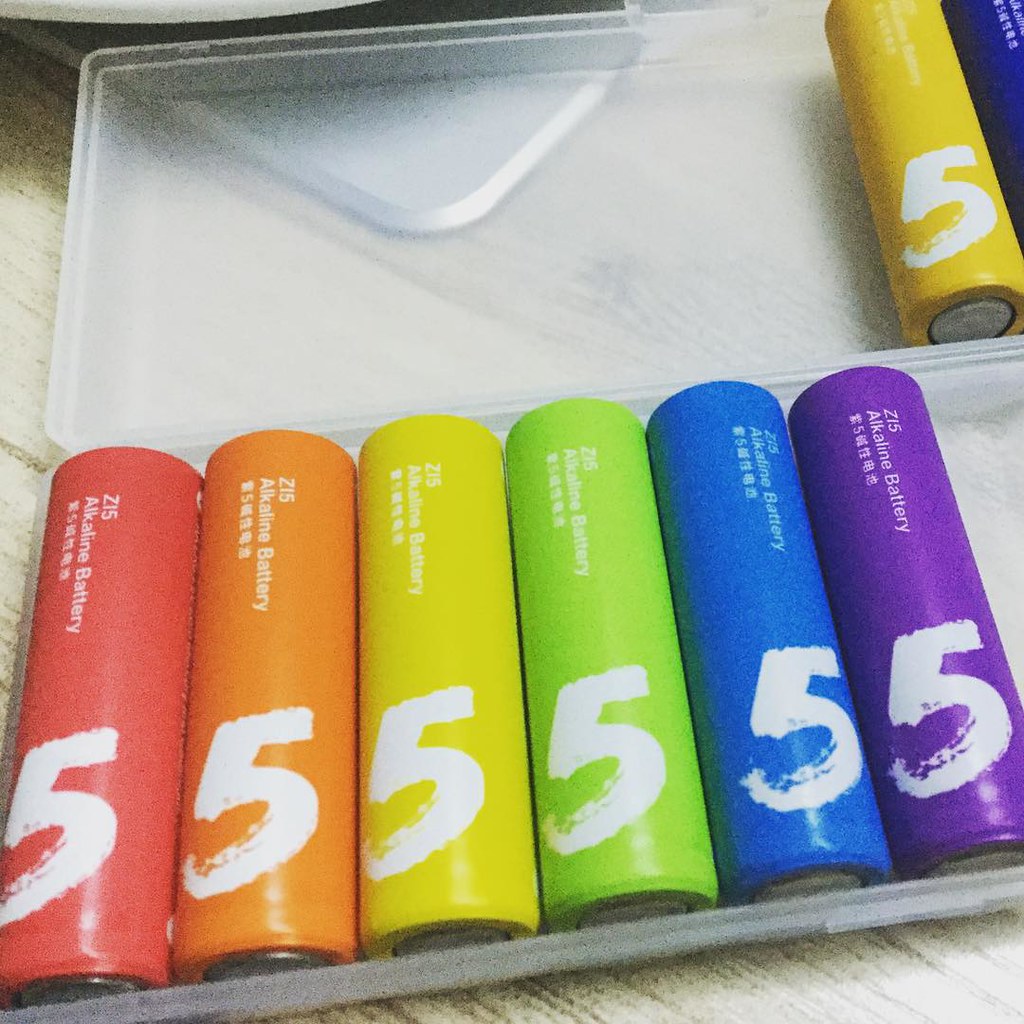The photograph showcases a set of six AA alkaline batteries housed in a translucent, white-colored plastic case. The batteries are arranged in a vibrant sequence resembling a rainbow: red, orange, yellow, green, blue, and purple. Each battery prominently features a large, white number "5" that appears to be painted in a brushstroke or chalk-like font, alongside the text "215 Alkaline Battery" and some Asian characters. One yellow battery has been removed from the case and is placed on top, revealing the case's open lid. The scene is set on a pale wood countertop, with a hint of a silver sink visible underneath. The vivid colors and chalk-like numbering on the batteries lend an initial impression that they might be crayons.